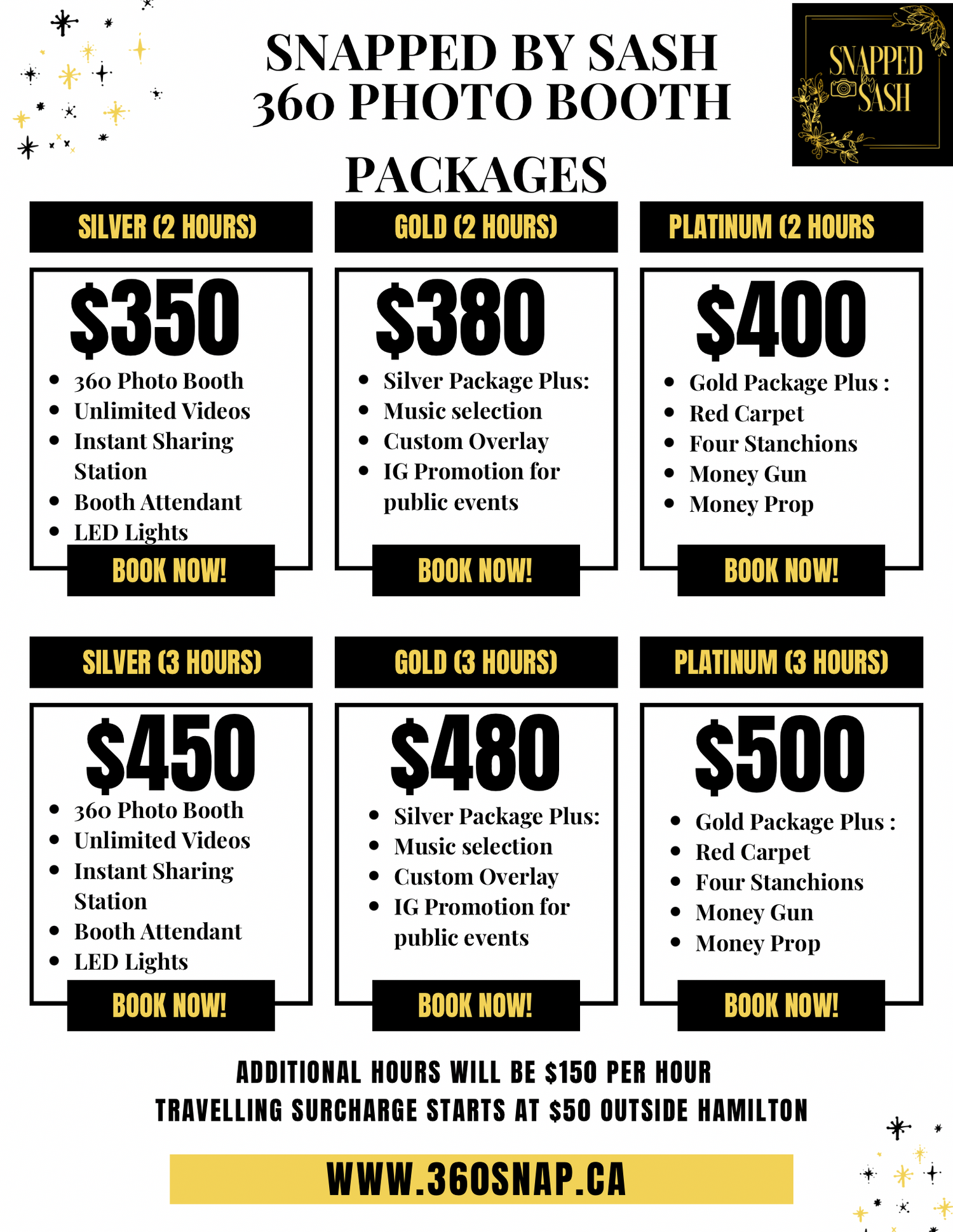The image is an advertisement for Snapped by Sash360 photo booth packages, featuring a sleek black and gold design on a white background. The top of the poster prominently displays the brand name "Snapped by Sash360 Photo Booth Packages." Below this, there are six packages outlined in individual boxes, each with a black title and gold text indicating the package names and details.

The packages are organized as follows:
1. Silver for 2 hours at $350, which includes the 360 photo booth, unlimited videos, an instant sharing station, a booth attendant, and LED lights.
2. Gold for 2 hours at $380, featuring all the silver package benefits plus music selection, custom overlays, and Instagram promotion for public events.
3. Platinum for 2 hours at $400, which includes all the gold package offerings and adds a red carpet, stanchions, and money gun props.
4. Silver for 3 hours at $450, offering the same benefits as the 2-hour silver package but for a longer duration.
5. Gold for 3 hours at $480, including all the silver package features plus the additional gold package benefits.
6. Platinum for 3 hours at $500, encompassing all the gold package features with the added luxuries of a red carpet, stanchions, and money gun props.

Each box includes a "Book Now" button and a list of package benefits. At the bottom of the advertisement, it mentions that additional hours can be purchased at $150 per hour and that a traveling surcharge starting at $50 applies outside of Hamilton. The website for booking is www.360snap.ca.